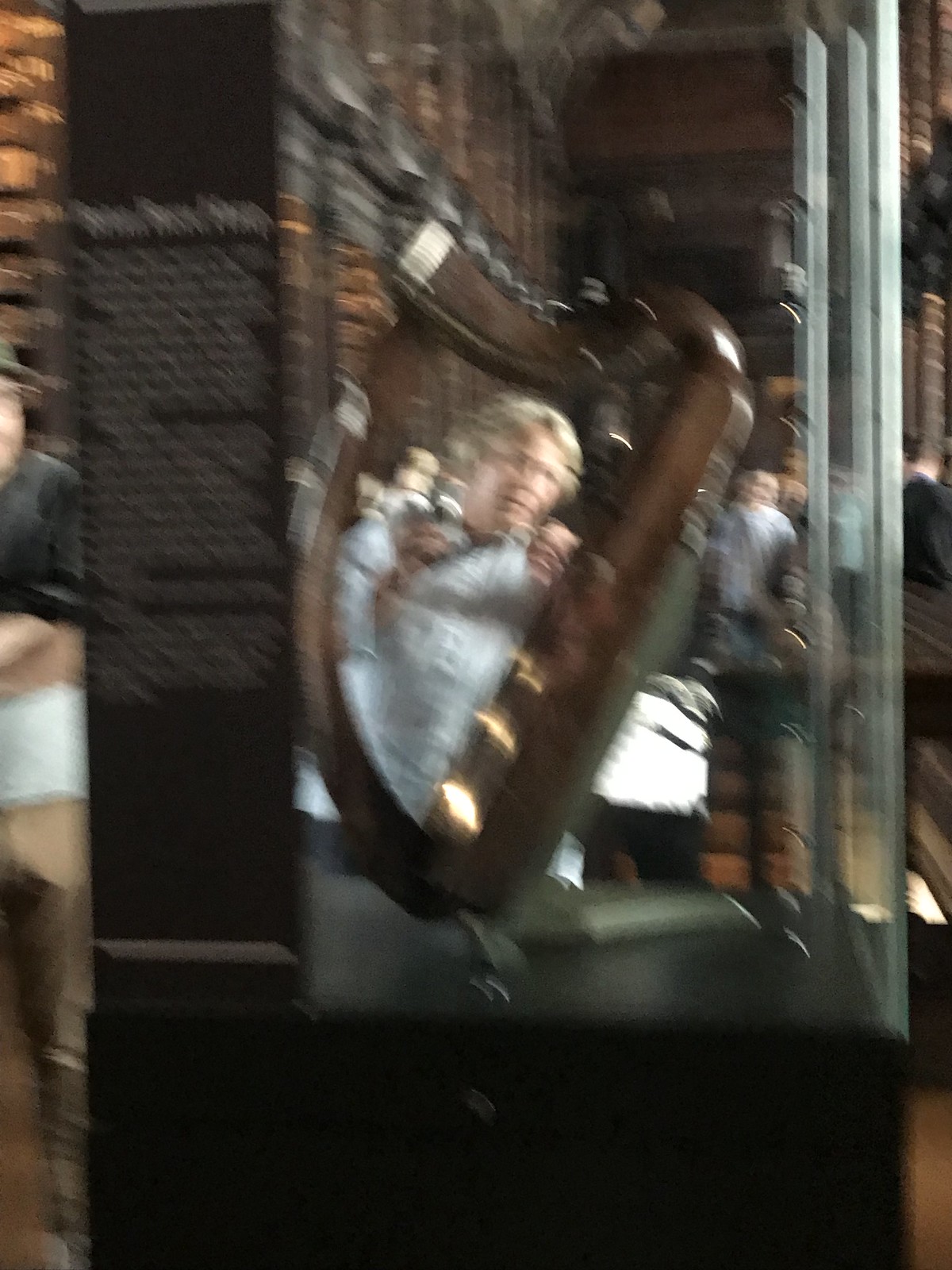A slightly blurred indoor photograph, likely taken in a museum setting, showcases a beautifully crafted object displayed within a protective glass case. The wooden item features elegant curves and has a rich, glossy walnut finish, hinting at its possible identity as a historically significant harp. The display case itself has a black base and clear glass sides, providing a pristine view of the object. Although the item's description on the side of the case is illegible due to the blur, one can infer its importance. Standing behind the display is a person with blonde hair, dressed in a light-colored top, intently observing the artifact. In the background, other visitors can be seen scattered throughout the facility, engrossed in their own explorations.